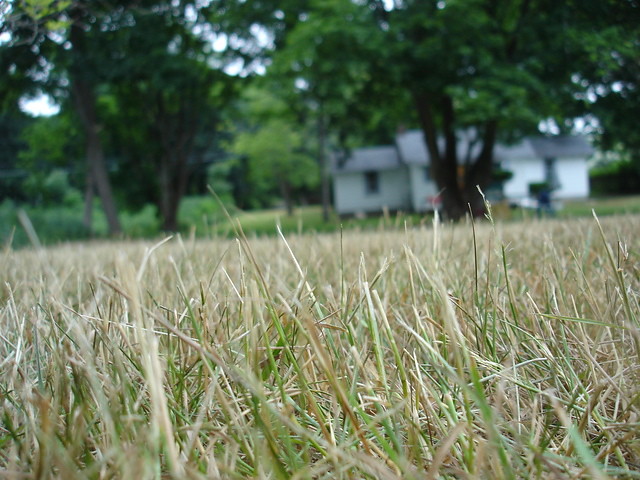The image is a close-up of mostly brown, dying grass with some green patches, indicating about 75% of it is dead. The grass, appearing short and slightly mowed, occupies the entire lower half of the image, suggesting a perspective close to the ground. In the blurred background, a white, single-story house with a dark-colored roof is surrounded by healthy, green trees. The scene is visibly bright with a blue sky, hinting at a sunny daytime, likely in the summer or late summer. Additional details include green shrubs to the left and possible seating or figures near the house, contributing to the cozy, nature-immersed setting.